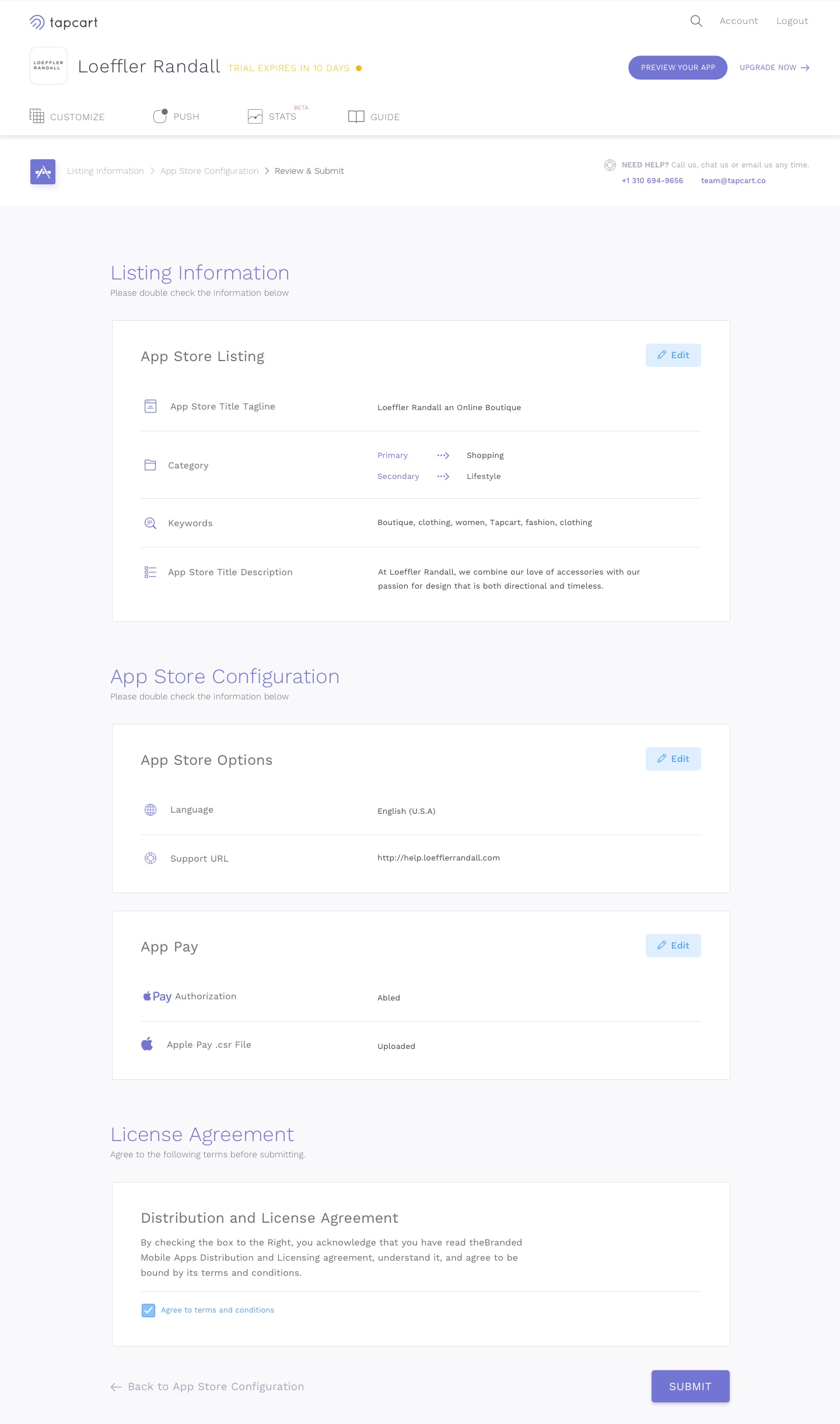This image, taken from an app store website, displays a user interface that allows app creators to list their applications. The page appears faint and has a pale white background with very light pink boxes containing the various options for customization.

At the top of the screen, the logo "TopCart" is faintly visible. Beneath it, there is a text that reads "Loffler Randall". Another button labeled "Preview Your App" is also at the top, suggesting a feature for users to review their app's listing before publishing.

The main content of the page includes several sections:

1. **Listing Information**: This section, titled "App Store Listing", allows users to edit their app's information—such as the category, associated keywords, tagline, and description—ensuring that the app is correctly listed.

2. **App Store Configuration**: Users can modify app store-specific options, including language settings and customer support details.

3. **Payment Options**: Under the "App Pay" section, users are able to edit the accepted payment methods for their app.

4. **License Agreement**: This section provides the terms for distribution and the license agreement associated with the app, which users can edit as necessary.

Overall, the faded appearance of this webpage may make it hard to read, but it depicts a detailed platform for developers to list and customize the description and configuration of their apps on the TopCart listing site.